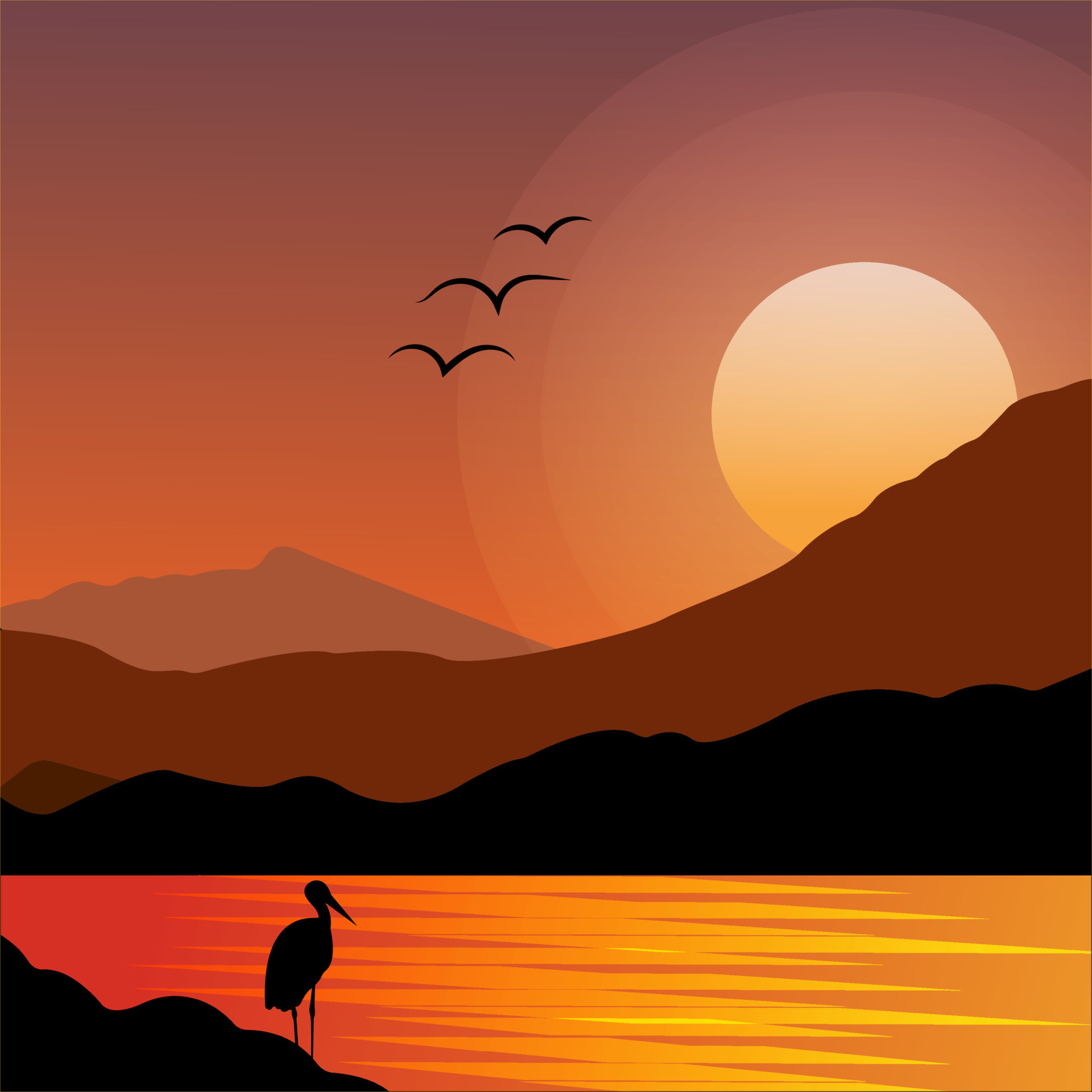The image depicts a minimalist painting featuring a striking palette of black, white, yellow, orange, red, and pink. The composition centers around a body of water that reflects a gradient sky transitioning from gold and beige to vibrant reds and darker oranges. In the lower left corner, black silhouetted rocks stretch from the upper left down to the center, with a solitary pelican perched on one of these rocks at the water's edge. The pelican, alongside three birds flying overhead, is rendered as a simple black silhouette. To the background, a harmonious blend of mountains in brown, light purple, gray, and black rises, with the largest mountain extending from the center left to the center right, partially overlapping a gray one. The dominant feature in the sky is a large circular sun setting behind these mountains, casting an atmospheric glow. The setting is clear and well-lit, with no additional text or numbers to distract from the serene, natural beauty of the scene.